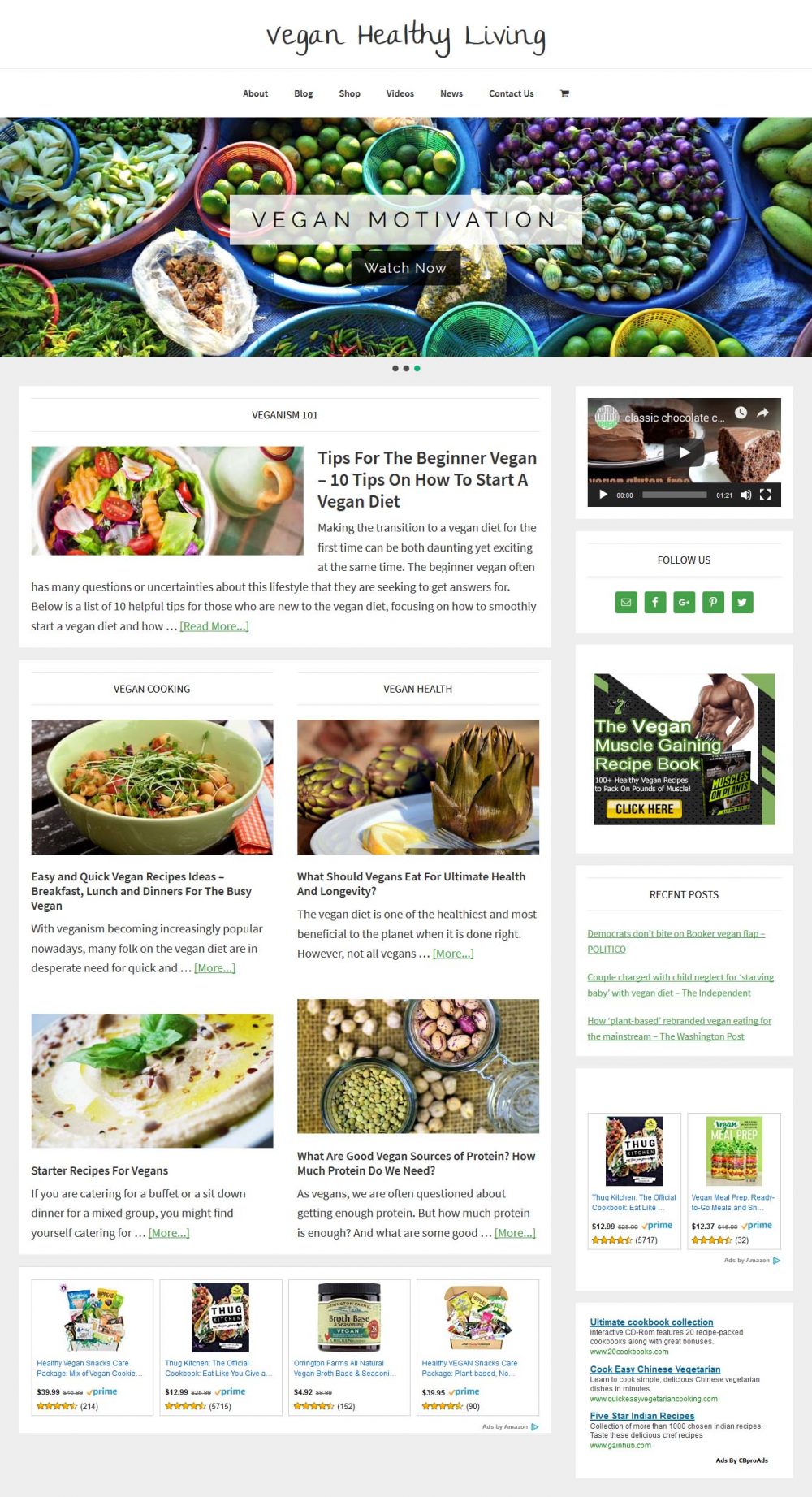This is a screenshot of a website called "Vegan Healthy Living." It features a clean, structured layout with a white navigation bar at the top, displaying seven tabs in black text: "About," "Blog," "Shop," "Something," "News," and "Contact Us." Also present is a black shopping trolley icon. Below the navigation bar is a large banner photograph. Centered on this banner is a white text box with black letters reading "Vegan Motivation," and directly beneath it, a black bar with white text stating "Watch Now."

The background image behind these text boxes displays an array of shallow bowls containing a variety of berries, vegetables, and spices, all meticulously arranged on a blue plastic sheet. The bowls come in different sizes, with some nested within others, reminiscent of a bustling market scene in India. 

Below the banner, the website features multiple news stories with photographs related to vegan cooking and health, including images of artichokes and salads.